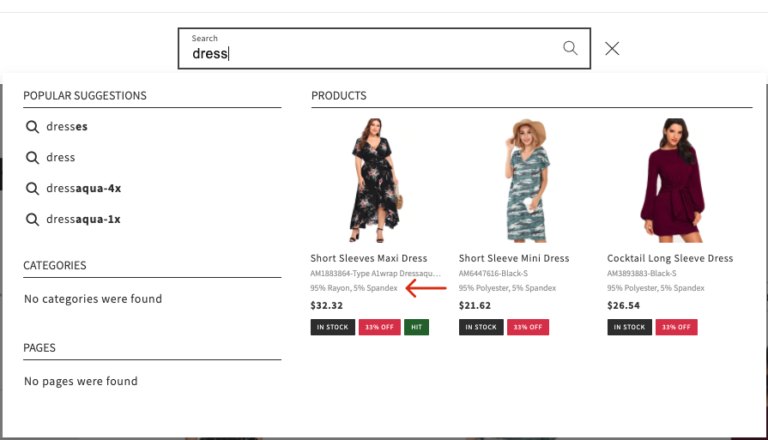The image is a screenshot from a clothing website. At the top, a search bar is highlighted where the user has typed in "dress." An 'X' button next to the search term allows for clearing the search. The product results display:

1. A short-sleeved maxi dress in black adorned with floral patterns.
2. A short-sleeved mini dress in a camouflage print.
3. A burgundy long-sleeved cocktail dress with a front tie, which falls just above the thighs.

Additionally, there's a section titled "Popular Suggestions" with search suggestions including "dresses," "dress," "dress aqua-4X," and "dress aqua-1X." Under the "Categories" and "Pages" headers, it indicates that no categories or pages were found.